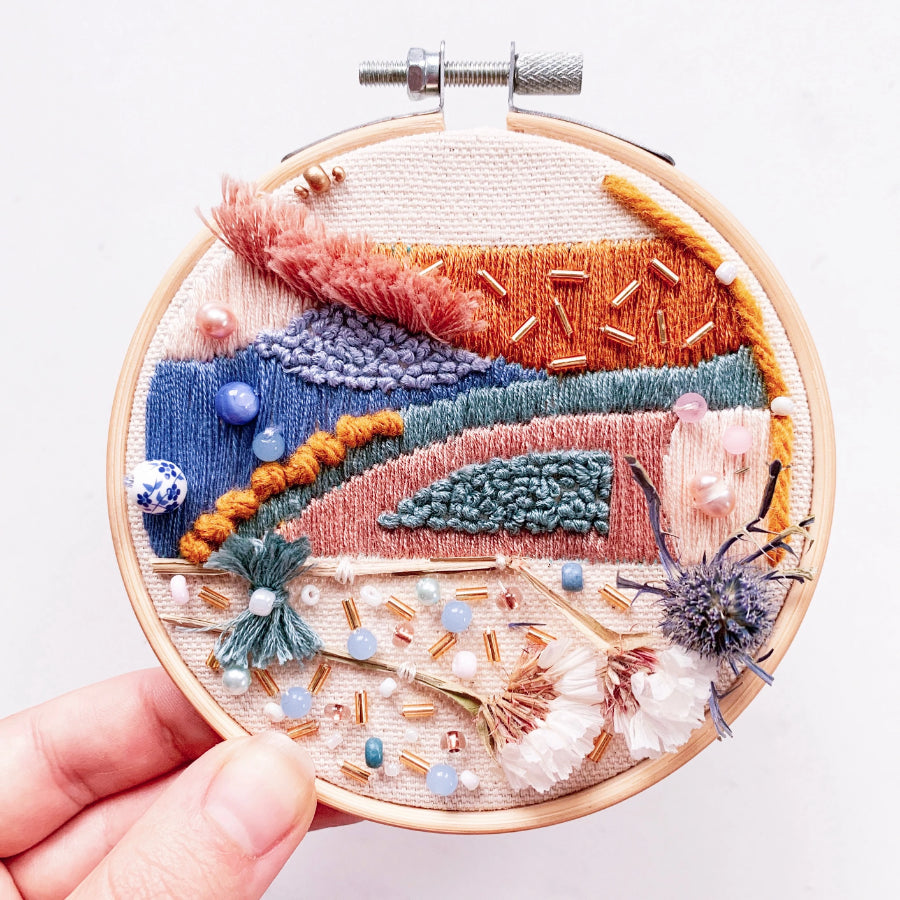This image features a person holding an intricately embroidered artwork, framed inside a wooden embroidery hoop. The background is pure white, highlighting the delicate details of the piece. The embroidery spans a variety of stitches, creating an abstract yet harmonious design. Among the featured stitches, there are satin stitches, chain stitches, knotted stitches, fan stitches, pearls stitches, and fringe, showcasing the embroiderer's extensive skill and creativity.

The color palette includes soft, pastel tones with threads in orange, lavender, blue, green, and pink. Prominent within the design are two white embroidered flowers, complemented by a mix of beads including lavender, copper, and various long beads. Additionally, the artwork incorporates elements like a silver bolt and screw, and an assortment of both blue and white beads with blue floral patterns.

The embroidery further includes rich embellishments: a rope looped on the right side, gold accents, and a bow-tie shaped stitch adorned with a white bead. The bottom section features a blend of white, gold, and blue beads against a light pink background. Overall, the design intermixes vibrant colors and textures, ranging from buzzy pinks and purples to brown, creating an ornamental piece that is both visually and texturally captivating.